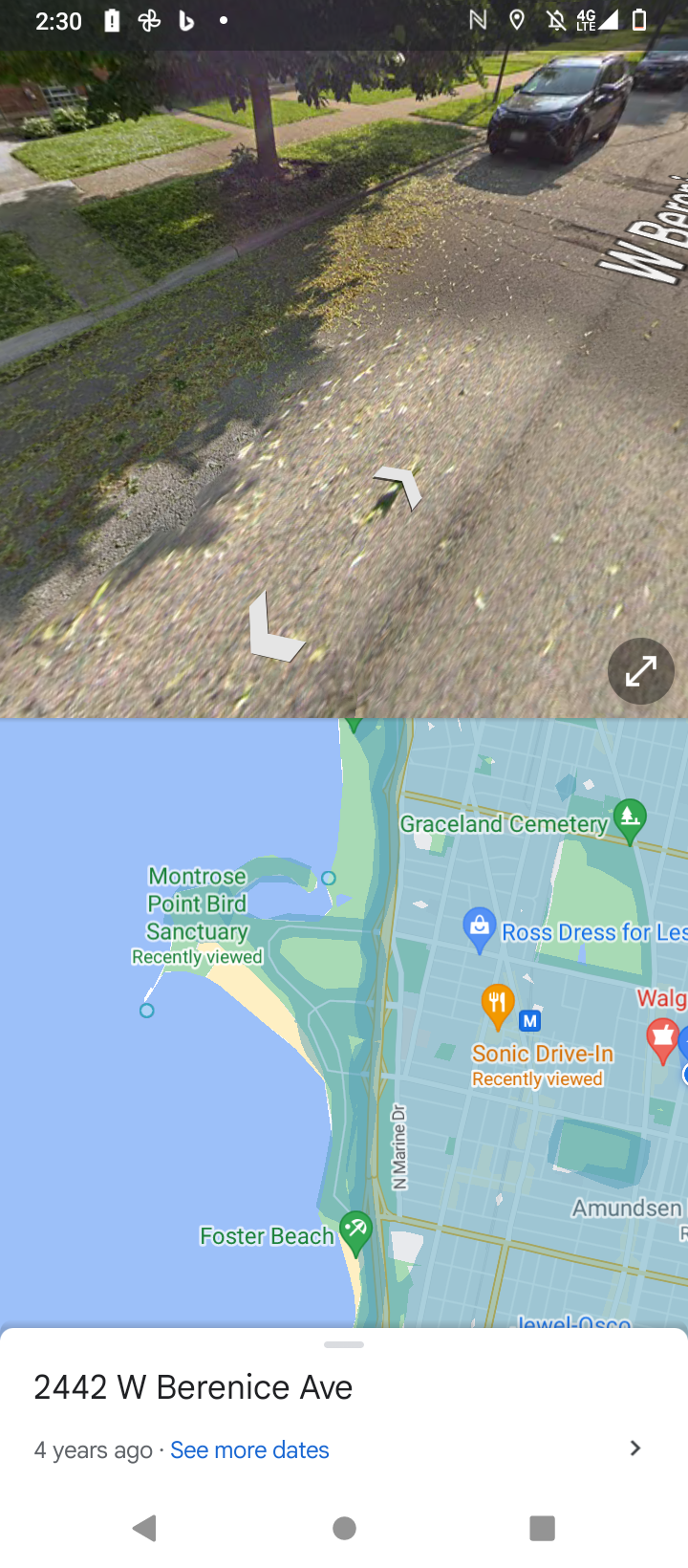This image is a detailed screenshot from a smartphone's navigation app, presenting both a split-screen view of a map and a Google Street View image. The upper part of the screen highlights a residential street scene from 2442 West Berenice Avenue, showing a paved road, green lawns, a sidewalk, and several cars parked on the curb. The street view offers a realistic perspective with the road running from the upper left to the upper right corner, bordered by trees and houses. At the top of the screen, typical smartphone indicators like the clock showing 2:30 PM, full battery status, and service bars are visible, confirming it's a mobile device screenshot. The lower part of the image displays a colorful digital map centered on Montrose Point Bird Sanctuary, with clearly marked features such as water bodies in blue, parks in green, and streets in light green. Additional points of interest like the Graceland Cemetery, Sonic Drive-In, and Walgreens are also visible. This comprehensive view suggests the user might be examining directions or planning a visit, with the address 2442 West Berenice Avenue and a timestamp of "four years ago" noted under the map.